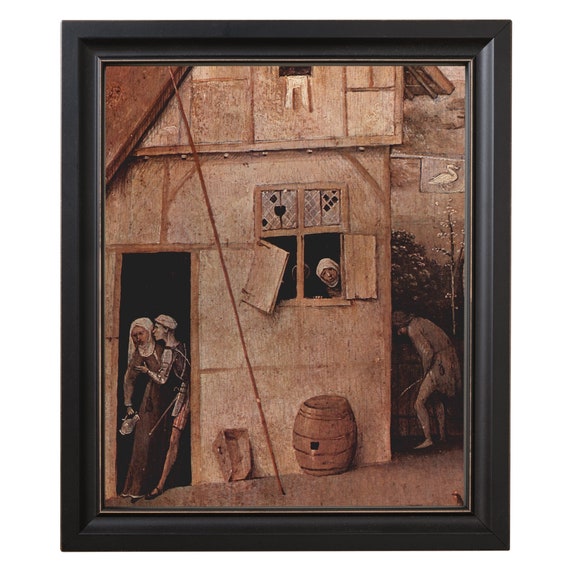This photograph captures an intricate painting framed in black, with an inner silver or white lining. The painting itself predominantly uses tan and brown hues, resembling a sepia-tone image. 

The central focus is a rustic house with a brown and beige facade. The house features a rooftop matching the brown color scheme and two windows with wooden shutters; one shutter is notably falling off. A woman in a white headdress peers out from one window. A flag adorned with a white swan hangs from the building, set against a tan backdrop. The background also includes greenery with brown and green stems and leaves.

In front of the house, a brown barrel sits beneath the window with faulty shutters. A figure clad in gray appears to be relieving themselves to the right of the house. Near the open doorway, inside which all is pitch black, stands a woman wearing a white scarf and holding a vase. Next to her is a man in a white hat, sporting a brown and white shirt, red and tan pants, and tan tights with black shoes.

Additional elements include a fallen box that is also brown, a horizontal black (or brown) line cutting diagonally across the painting, and a ground surface that is a grayish-tan color. Despite the muted and earthy color palette, the scene is teeming with details, from the broken glass in the windows to the vivid attire of its characters.